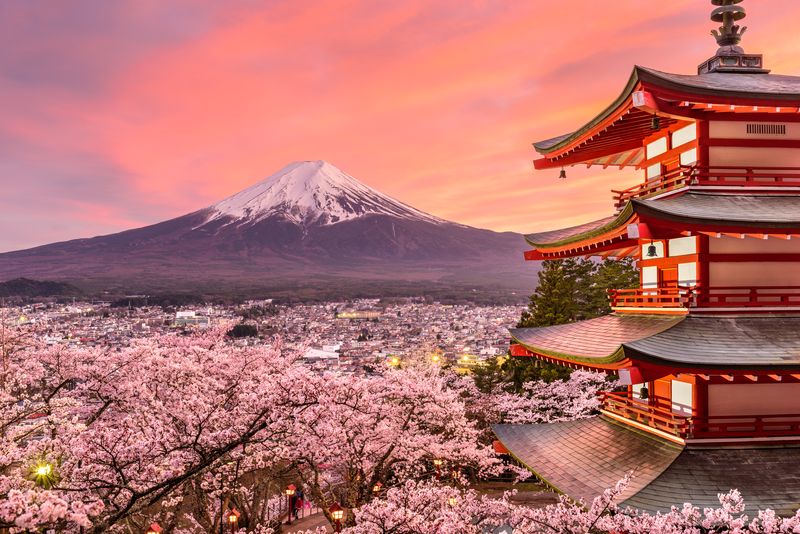The image captures a picturesque scene in Japan, intricately detailed and brimming with cultural elements. Dominating the right side of the rectangular frame is an Edo-period imperial castle, distinguished by its four connected tiers. Each tier is adorned with gray shingled roofs and red wooden beams, complemented by small wooden rooms with red doors. Intricately designed railings and vents, and bells on each level are noticeable. An evergreen tree stretches up near the castle, reaching almost to the third level. 

Surrounding the castle, cherry blossom trees are in full bloom, signifying springtime. Red lanterns hang among the trees, casting a warm glow that enhances the evening ambiance suggested by the vibrant sunset sky transitioning from purple to orange-pink hues. In the background, a majestic snow-capped mountain stands tall, framed by the bright sunset sky. Beneath the mountain lies a sprawling cityscape with numerous tiny, illuminated buildings, adding depth to the image. The scene is a harmonious blend of nature, traditional architecture, and the subtle indications of a bustling city under a beautiful dusky sky.